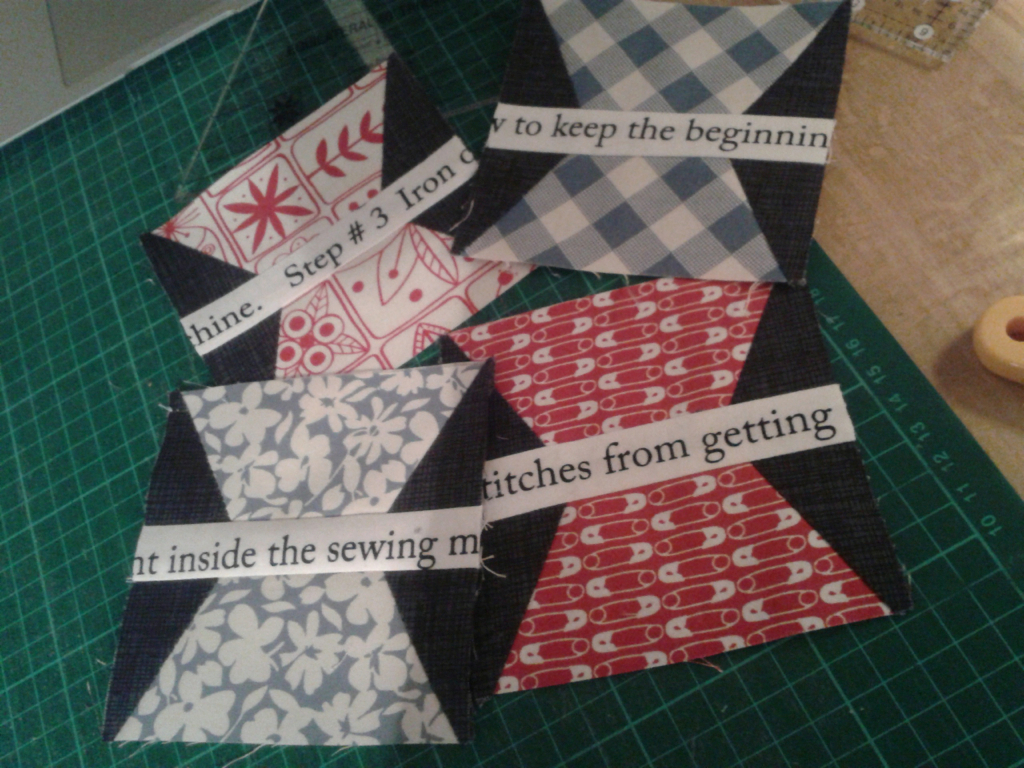This detailed image captures a sewing workspace featuring various sewing materials and fabrics arranged on a light tan wooden table. Prominently displayed is a large green measuring ruler with numbered white squares, labeled from 10 to 18, helpful in precise cloth measurements. Surrounding the ruler are multiple fabrics and instructional cards, each seemingly part of a sewing project. One card features a white fabric with red flowers and the words "Step 3 Iron," while another displays blue fabric with white flowers and the label "Inside the Sewing." A gray fabric card within a sewing machine showcases steps for stitching, including phrases like "stitching from getting" and "to keep the beginning." The entire setup is placed on a green background cutting board, marked with grids and numbers, ideal for arts and crafts measurements. The scene suggests an organized, detailed step-by-step guide to creating a sewn item, alluding to a structured, creative sewing project in progress.